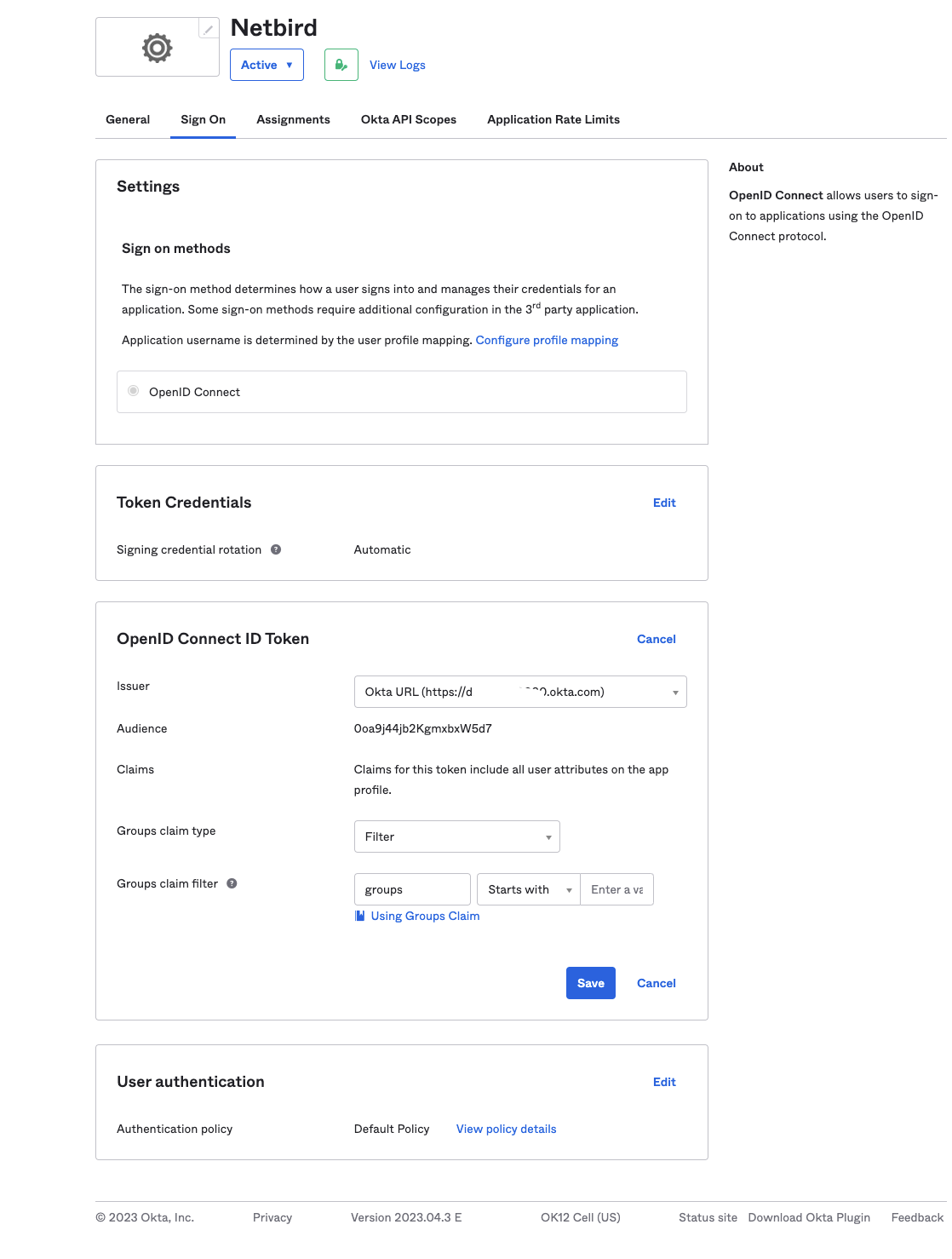The image features a detailed interface layout with a predominant white background. At the top, there is a gray gear icon beside the text "NetBird" in black. Below that, in a green box with a key icon, "Active" is displayed in white text. To the right of this box, the words "View Logs" are highlighted in blue.

Underneath, "General" is written in black text, accompanied by a blue underline. The sections "Assignments," "OKTA API Scopes," and "Application Rates" are listed below.

A thin gray line horizontally divides the interface, followed by a rectangular box containing "Settings" in black text. The description within this box details "Sign-on methods," which explains the process and various requirements for user sign-in and credential management. It mentions the need for additional configuration in third-party applications and specifies that the application username is determined by the user profile map, followed by a blue "Configure Profile Map" link.

The next section deals with "OpenID Connect" in black text. Following this, there is another rectangle outlined with "Token Credentials," detailing "Sign-in credential rotation" set to "Automatic." A blue "Edit" link is also present.

In a subsequent rectangle, the text "OpenID Connect ID Token" is displayed, followed by categories such as "Issuer," "Audience Claims," "Group Claims Type," and "Group Claims Filter." It specifies the OKTA API URL and notes that the token includes all user attributes on the app profile, with instructions to filter groups starting with a specific prefix. The text cuts off at "Enter a VA," and a blue "Use Groups Claim" link is visible.

Finally, at the bottom, a blue rectangle contains the word "Save" in white text, with "Cancel" in blue text adjacent to it.